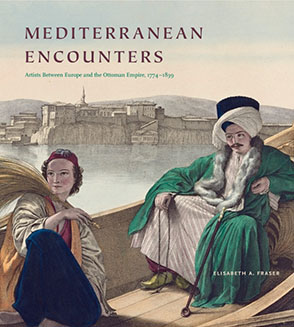This detailed book cover of "Mediterranean Encounters" by Elizabeth A. Fraser illustrates a vivid scene likely set during the Ottoman Empire between 1774 and 1839. The foreground features two individuals in a boat, one female and one male. The woman on the left, dressed in white and red attire with blue pants and a yellow satchel slung over her right shoulder, appears to be holding a broomstick or possibly wheat or grain. The man on the right is adorned in a green jacket over a white inner layer, with a white head covering and long, striped robe. His outfit is completed with striking gold boots, and he has long hair and a mustache. The backdrop includes a gray and peach-hued sky with hills, possibly portraying the cityscape of Istanbul, Turkey. This captivating imagery sets the scene for a scholarly exploration of interactions around the Mediterranean during this historical period.